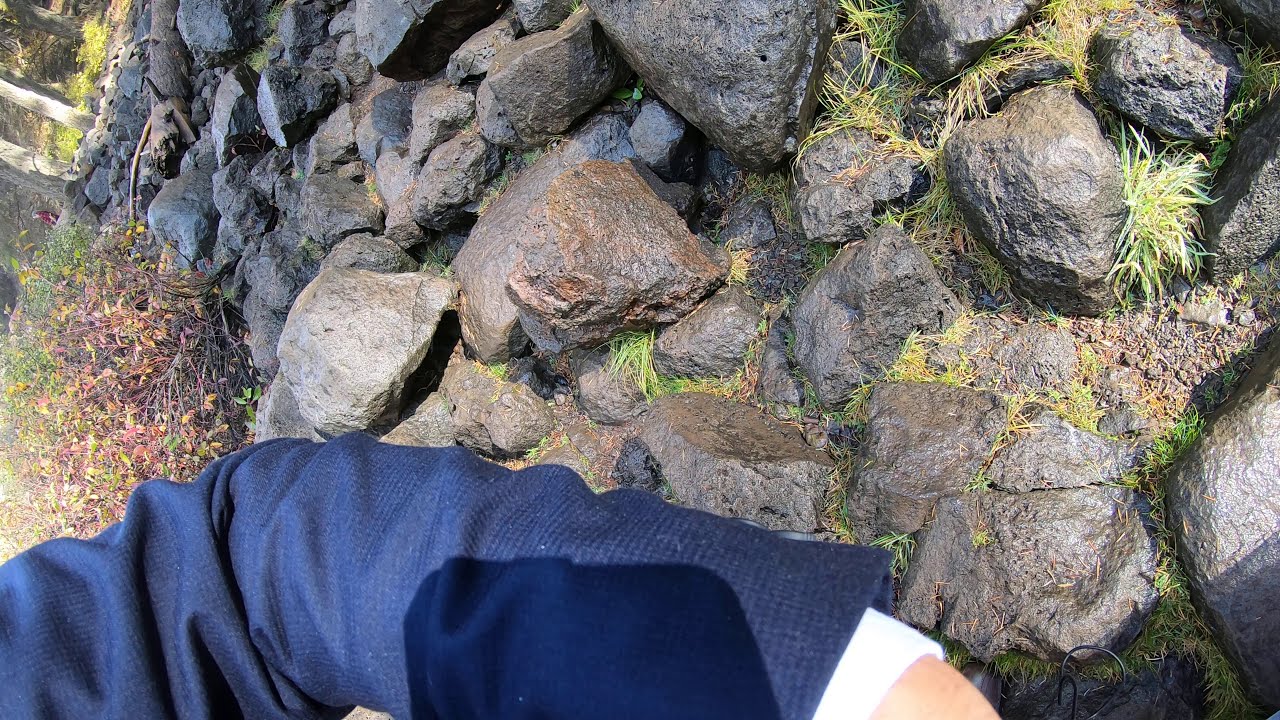The image is a slightly tilted photograph taken outdoors, featuring a large rocky formation primarily consisting of dark, gray, black, and brown boulders with a relatively shiny texture. Grass grows sporadically among the rocks, with some pebbles interspersed in between. To the left, there are visible shrubs and dry leaves lying on the ground, as well as some twigs with leaves, possibly indicating the presence of a bush. In the background, the trunks of a couple of white trees and additional trees beyond can be seen, suggesting a wooded area. A notable detail is the forearm of the photographer, clad in a blue sleeve with a patch near the end, and a white shirt peeking from underneath. The arm covers a portion of the lower part of the image, extending from the forearm to the wrist and partially revealing the skin on the top of the hand. This arm positioning and the tilted orientation give the impression that the photo was taken accidentally.